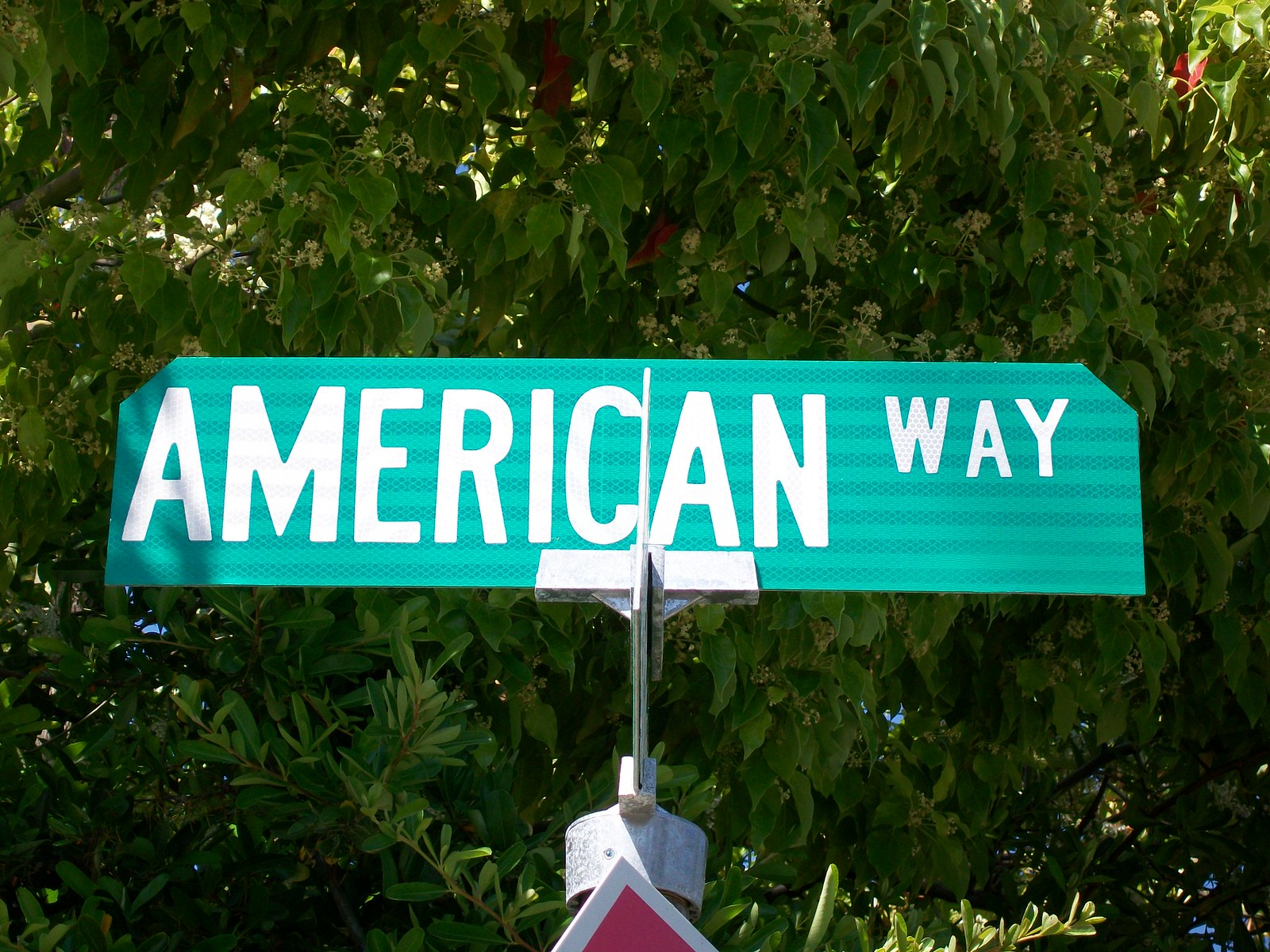An up-close photograph showcases a street sign that reads "American Way" in large, bold block letters. The word "American" is prominently displayed, while "Way" appears slightly smaller but equally bold. The sign itself is running horizontally with slightly truncated corners at the top, giving it a unique shape. Mounted on a sturdy circular metal post, the "American Way" sign intersects another street sign going in the opposite direction. Below the "American Way" sign, a red sign with white trim, pointed at the top, is partially visible. In the background, a lush, flowering tree with vibrant red blooms or butterflies adds a pop of color, contrasting with the green foliage, creating a picturesque urban scene.